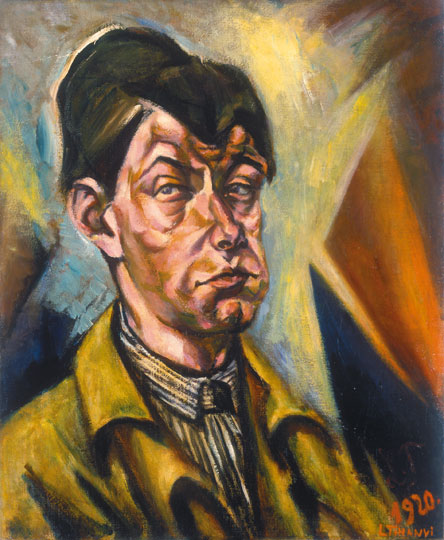This painting, dated "1920" with the partially legible name "L-T-H-N-V-I" at the bottom, depicts a young man with brown hair, possibly wearing a small black cap that blends with his hair. He appears to be deep in thought, his expression serious with a frown, pursed lips, and eyes glaring intensely. His facial features are rather wrinkled, giving his face a crumpled, textured look like a caricature or a cubist interpretation. He wears a mustard yellow jacket over a black and white striped shirt. Behind him, a complex background features a seven-pointed white star with jagged tips, interspersed with triangles of orange and blue, atop a backdrop of yellow, orange, and blue splashes, possibly suggesting city lights.